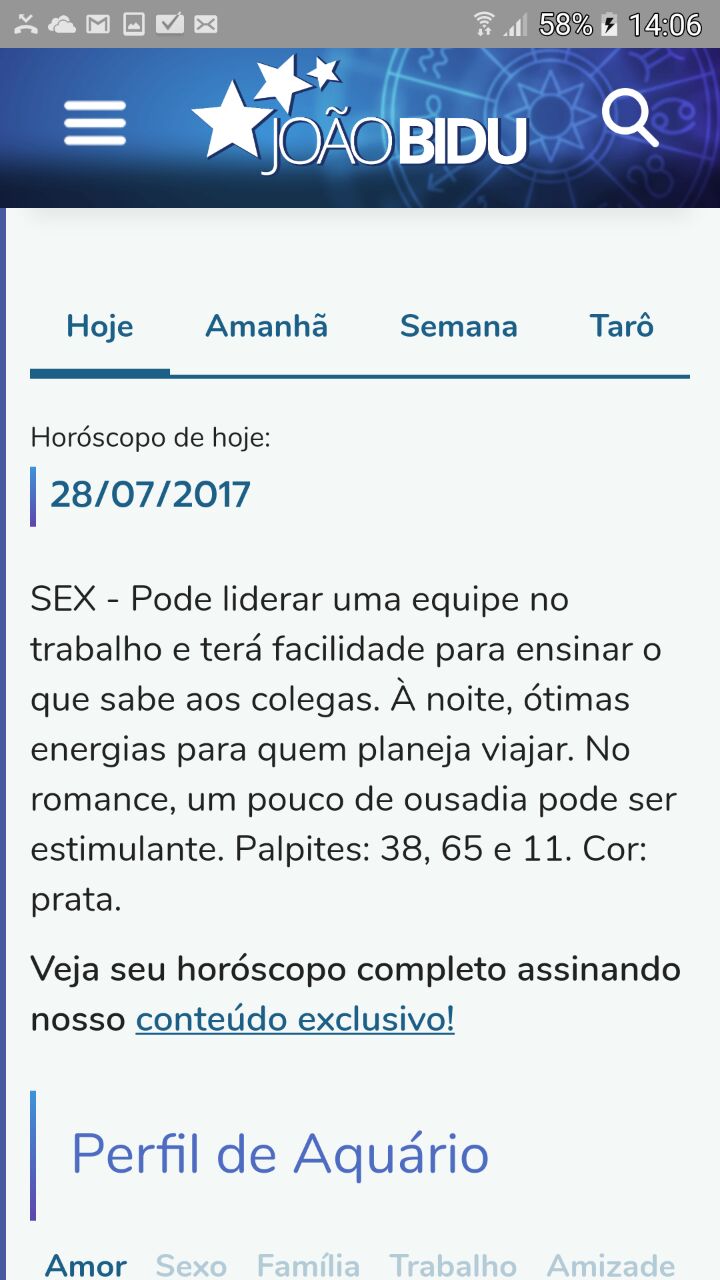This is a screenshot taken from an Android device showing an in-app horoscope from Joao Bidu, dated July 20th, 2017. The phone's interface reveals a battery status of 58% and the time as 14:06, indicated on a gray bar across the top of the screen with additional system icons present. The app itself has a header with a blue and purple gradient background, featuring a semi-transparent astrological chart and three white stars. The header includes a menu icon on the left and a magnifying glass search icon on the right. Below the header, there are four tabs with menus written in Portuguese. The main content of the app is displayed on a light gray background, with key details such as the horoscope category "amor" (love) highlighted, and links within the text are marked in teal. The app appears to provide horoscope information digitally in black text on a white background, with blue accents for dates and other key elements.